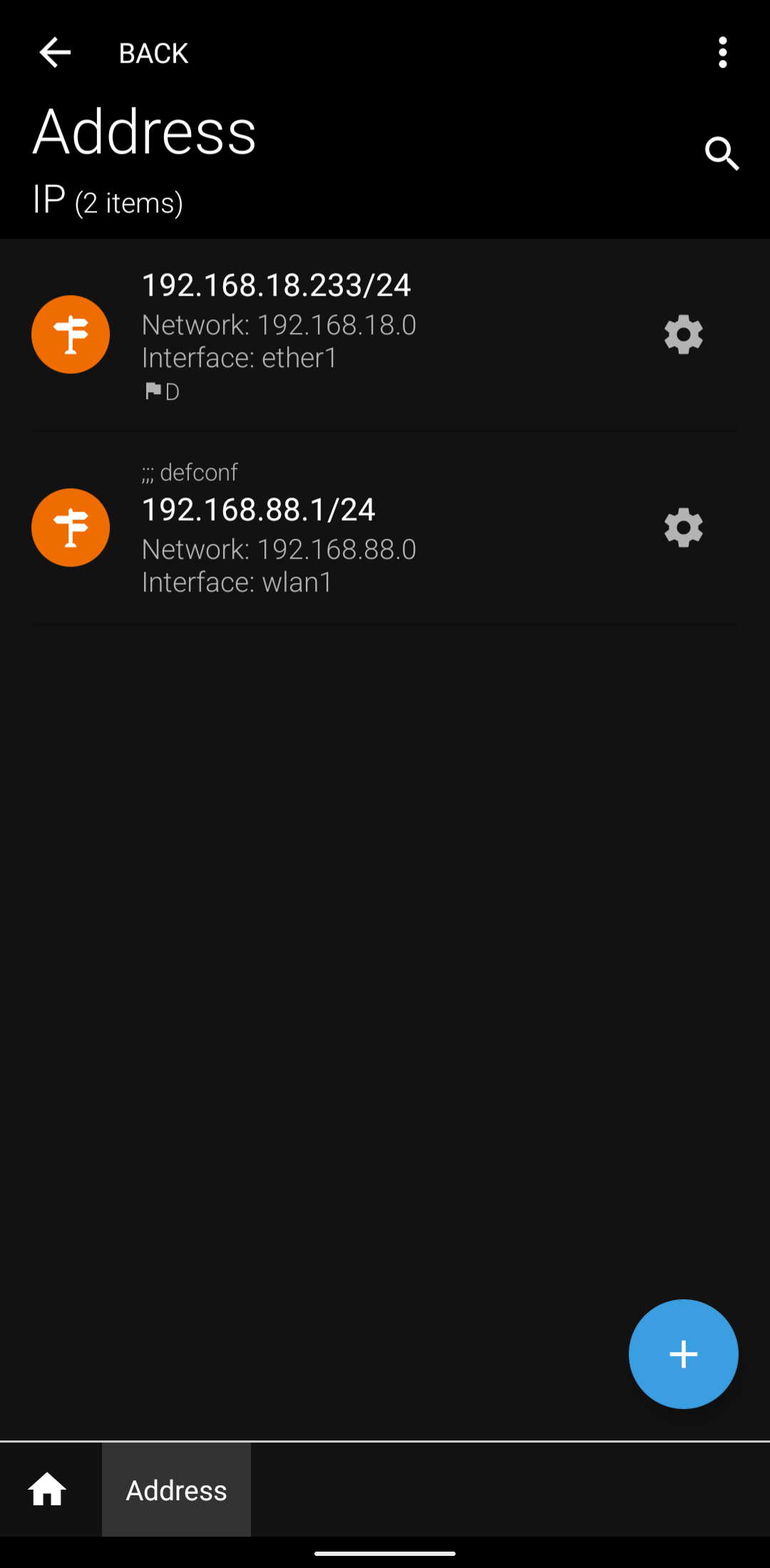**Detailed Caption:**

This image is a screenshot from a smartphone, predominantly dark-themed with significant white text and logos in orange and purple. At the top left corner, there is a left-facing arrow labeled "Back," followed by three vertical dots positioned to the right, indicating a menu option. Below these, text labels read "Address," accompanied by a magnifying glass icon (search function). 

Immediately below, the text “IP” appears, accompanied by the note “(two items)”. 

Below this section, there are two identical orange logos. Each logo resembles a post with three street signs—two signs point to the right, and one points to the left. To the right of these logos are segmented IP address-like sequences, specifically "192.168.18.2334.24," and beneath that, the notation “Network” followed by "192-168-18-0" and “Interface: either one”. 

Further down, there is a flag icon with an uppercase “D” next to it and a settings gear icon to its right. Below this setup is the same orange logo (a circle with a stand resembling a post with three street signs). Above this logo, in capital letters, is "DEF CON." 

This section again lists IP addresses, specifically "192.168.88.14-24," followed by "Network 192.168.88.0" and “Interface: WLAN number one”. Adjacent to this text on the right is another settings gear icon. 

At the very bottom, there is a noticeable blue circle containing a white plus sign. The screen’s footer exhibits common navigation icons: a home button and "Address," with the current screen highlighting “Address”.